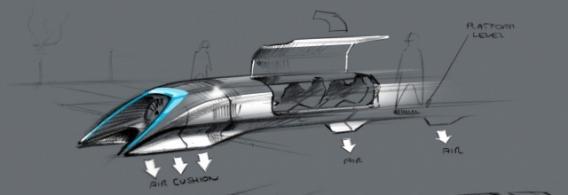The illustration is a detailed concept art sketch of a futuristic, high-speed train prototype reminiscent of a bullet train, possibly akin to the Hyperloop design from SpaceX or Tesla. The entire image is predominantly in black and white, with intricate pencil markings and hints of ink or chalk detailing. The train features a distinctive front that is shaped like an upside-down horseshoe or a hair clipper guard, bordered in teal/blue. It has two sharp, tapering ends and an identifiable sleek design that emphasizes aerodynamic efficiency.

Labeled annotations provide schematic insights, such as three arrows pointing down from the front labeled "air cushions," suggesting the train's floating mechanism. A fly-out view reveals the interior passenger cabin, designed with vertically opening doors and showcasing multiple seats. The sketch includes additional figures around the train, along with a small scene in the back left featuring a tree and a sidewalk, enhancing the environmental context of the futuristic setting.